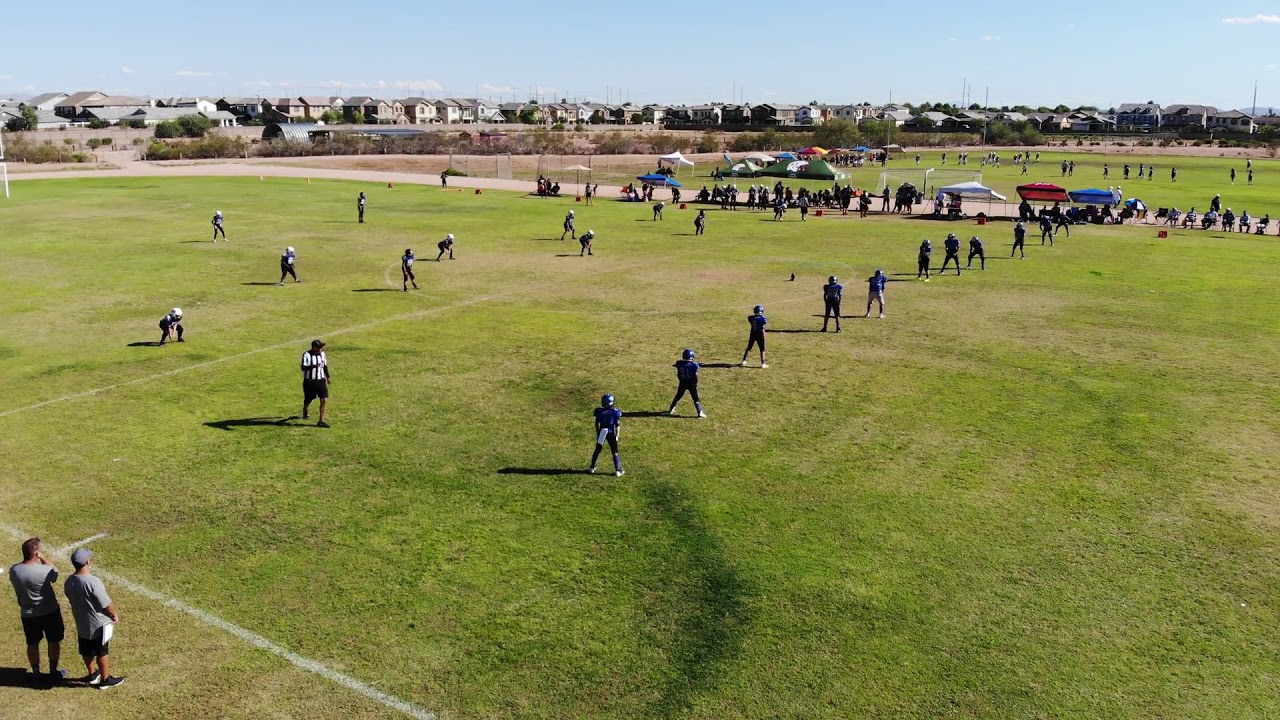The photograph captures an outdoor American football game during a sunny day with a clear blue sky. The scene is centered on a green football field, though the grass appears ragged in some patches. The image shows two teams lined up for a kickoff, with the team on the right side wearing blue shirts and blue helmets and the team on the left side in black shirts with silver or black helmets. A football rests on the field, ready to be kicked.

Adjacent to the sidelines in the bottom left corner, two men, presumably coaches, stand in gray t-shirts and dark shorts. Positioned more toward the center left, a referee in black shorts and a white and black striped shirt is visible.

Spectators populate the far side of the field, seated on benches and under umbrellas or canopies. Behind them runs a path or road, beyond which another football game is in progress on a separate field dotted with more tents and pavilions.

In the distant background, a suburban landscape emerges with a line of houses, dirt patches, and scrub. This detailed depiction showcases the bustling activity and community involvement on a serene, sunny day at the football fields.